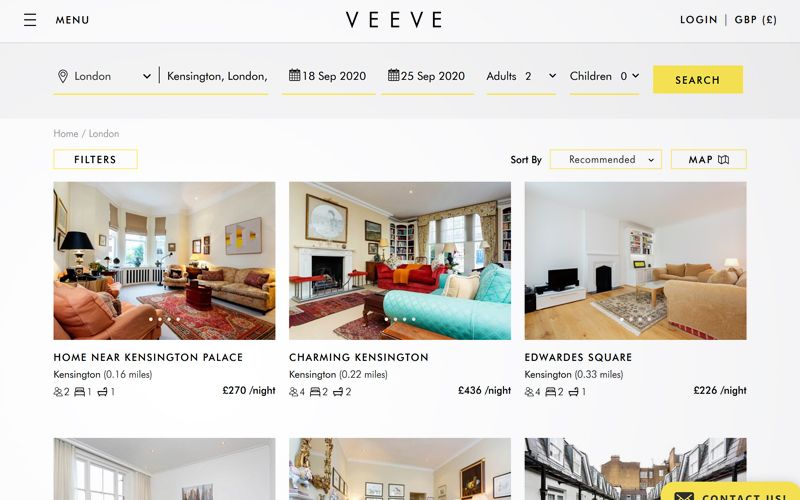The image features a user interface design against a very light purple background. At the top of the screen, three small horizontal black lines flank a centered section that contains the words "Menu" and "VEVE." To the right, there's a sequence including "Login," a thin vertical line, "GBP," and a small sign icon with the text "London." This is enclosed within a purple box, accompanied by a dropdown arrow and the words "Kensington, London," along with the date range "18th of September, 2020 through 25th of September, 2020." Below this, details show "Adults 2" with a dropdown and "Children 0" with another dropdown, followed by a prominent yellow search button. This entire section is underlined in yellow.

Further down, the background continues in light purple, organized into sections labeled "Home" and "London," alongside a yellow "Filters" button. There are options to sort, with two yellow buttons labeled "Recommended" and "Map." The visual content includes several room listings: 

1. An aesthetically pleasing room titled "Home near Kensington Palace" priced at £270 per night.
2. A room labeled "Charming Kensington" at £436 per night.
3. Another room named "Edward Square" costing £226 per night.

Additionally, the bottom of the image shows partial views of three more room pictures.